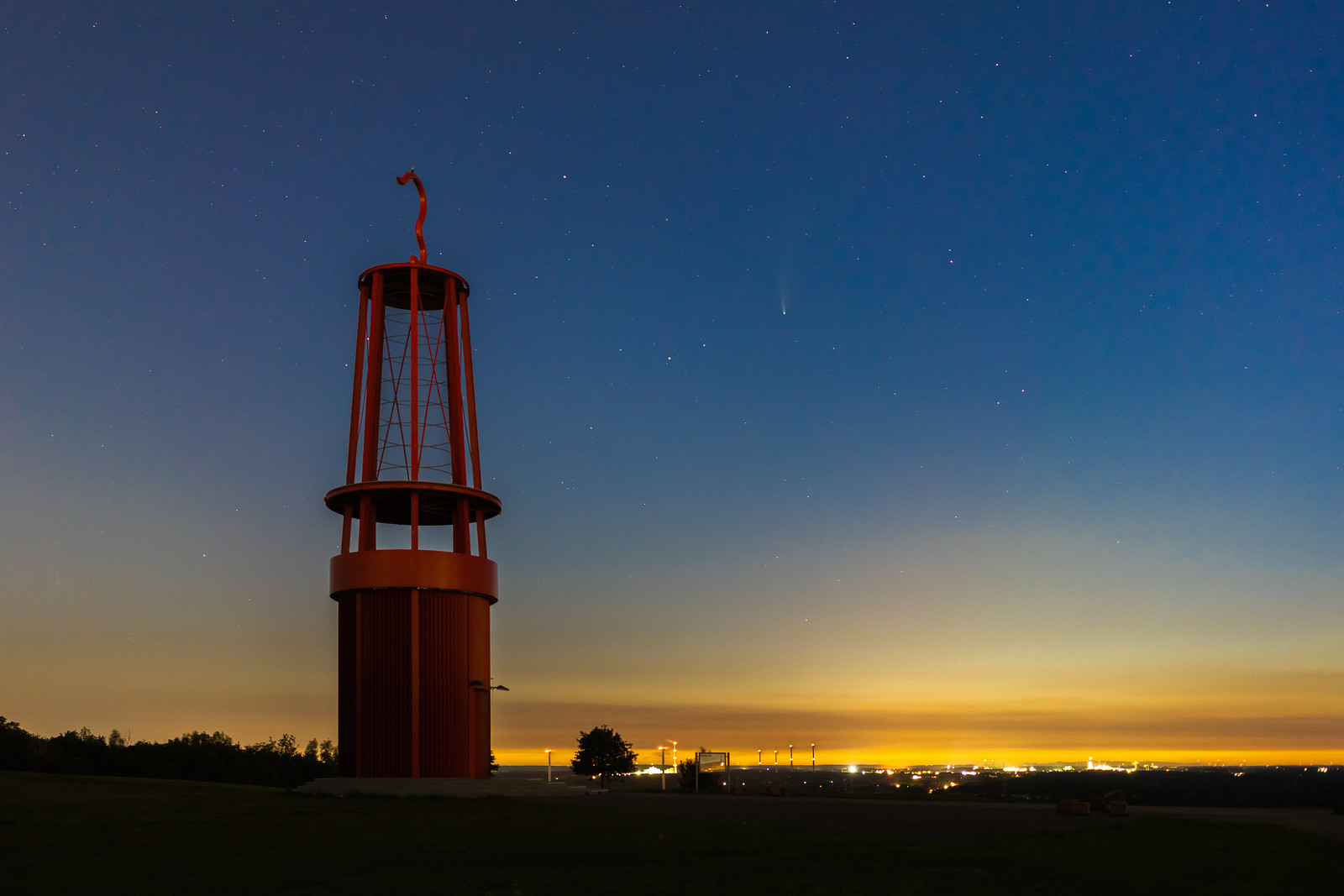A beautifully captured rectangular photograph taken outdoors at sunset showcases a stunning evening sky. The upper portion of the image is dominated by a deep, dark blue sky, accentuated by several twinkling stars. Along the horizon, a vibrant and fiery orange-yellow glow marks the sunset, illuminating the scene with its warm hues. Below this horizon, a populated area comes alive with the lights of various structures and buildings, including some streetlights, creating a sense of bustling life against the twilight backdrop.

In the foreground, to the left, stands an intriguing large red structure. It features a solid, round base that extends halfway up, transitioning into a framework of red beams. A solid disc-like element intersects through the middle of these beams, adding to its complex design. The apex of the structure incorporates a distinctive, large hook-like shape. The exact purpose of this structure remains unclear, but its bold presence and unique form draw the viewer's attention, adding depth and curiosity to the overall scene.